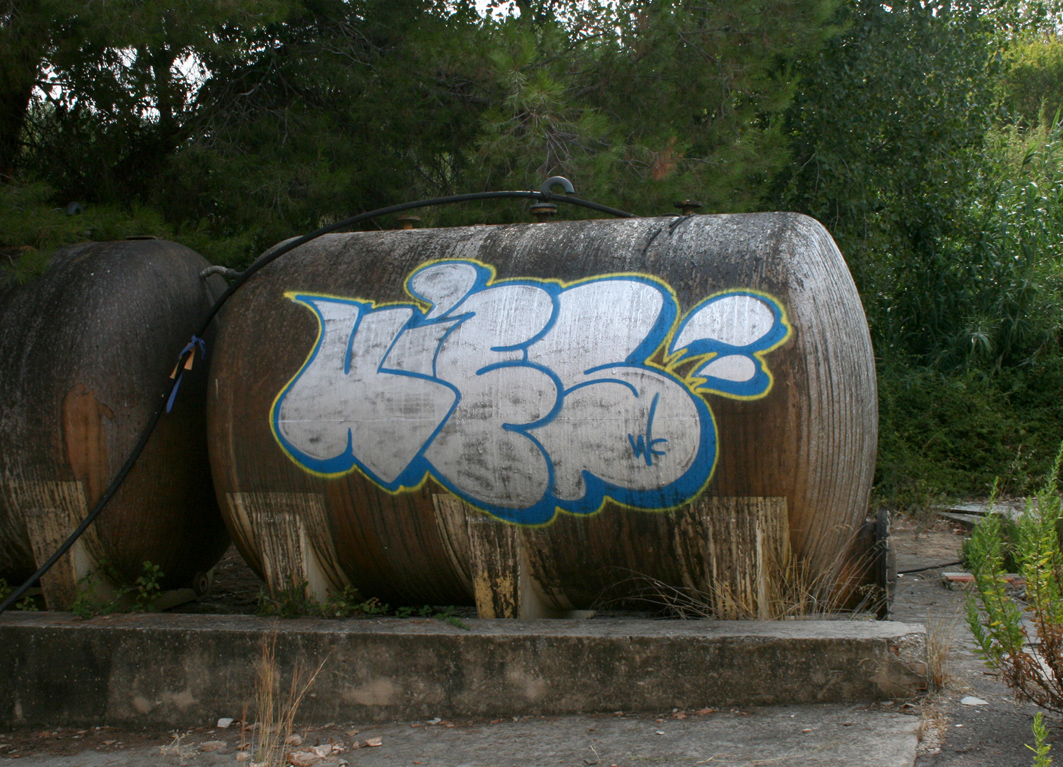In this detailed photographic image set outdoors in a forest during the daytime, a large, rusted brown cylindrical tank, resembling a propane tank, stands prominently on a concrete slab on a paved area. The tank showcases vibrant graffiti art, featuring white paint with bright blue and yellow outlines. The graffiti seems to depict an abstract representation that can be interpreted either as the letters "L-E-B" or a stylized image of a woman with discernible breasts, cheeks, and an enigmatic flow of water, accompanied by a face or a thought bubble. Mounted securely on its base, the tank also has a black hose running vertically behind it. To the right, a small plant and shrubbery add to the rich greenery of the background, where dense trees cast deep shadows but allow specks of daylight to filter through. This creates a juxtaposition of the rusty industrial element against the lush and shadowy forest backdrop.